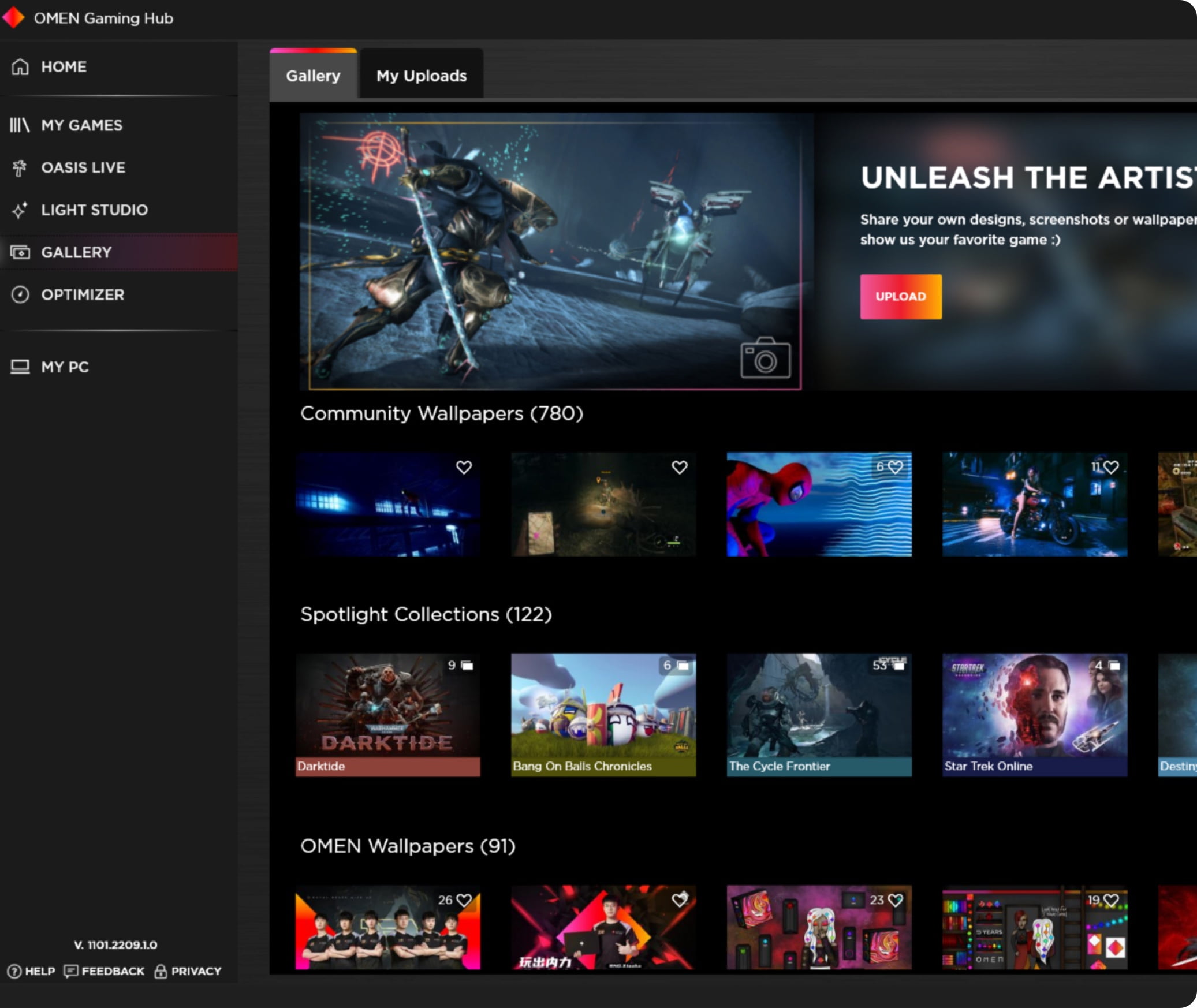The image features a sophisticated gaming interface layout. At the top left corner, there is a red diamond-shaped logo with a subtle white hue near its right tip, accompanied by the word "OMEN" in bold white capital letters. Directly beneath it, "GAMING HUB" is also displayed in white capital letters. 

On the left side, there is a vertical menu set against a black background. The first icon is a home symbol outlined in light gray, labeled "HOME" in white capital letters. Following this, a bright gray divider line is visible, fading towards the edges. The subsequent menu item features three white lines, one of which is slanted, accompanied by the text "MY GAMES" in capital white letters. The next icon resembles a wand, labeled "OASIS LIVE."

Following this is an icon featuring a sparkle with a dot in the upper right corner, marked "LIGHT STUDIO" in capital letters. Next on the list is an icon depicting an image overlapping another box, labeled "GALLERY." The subsequent option shows a circle with a dot in the center, labeled "OPTIMIZER." Another fading divider line follows this, with the final menu item displaying a computer icon labeled "MY PC."

On the right side of the interface, there is a large graphic featuring a robotic figure holding what appears to be a lightsaber in its right hand. In the upper right corner of this section, there is a neon red spaceship-like shape. The border surrounding this graphic transitions from light gray to yellow to pink. In the background, another spaceship or animatronic figure is partially visible on the right side. Overlaid in this section, the white text "Unleash the artist" is present but cut off after the letter "s."